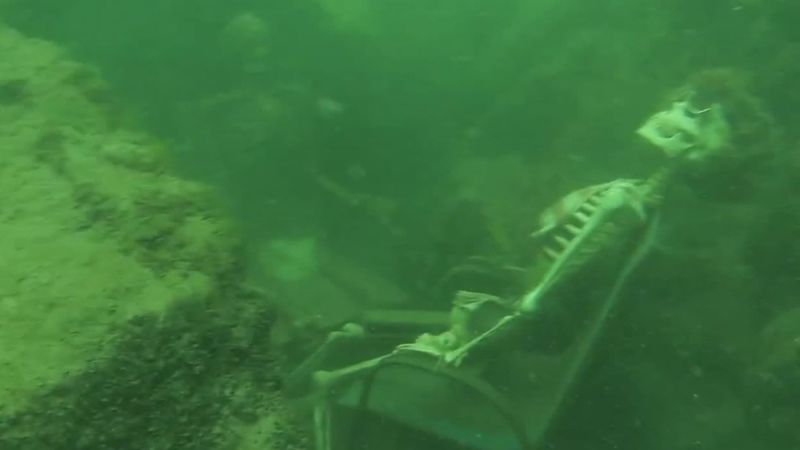This underwater photograph is enveloped in a green murkiness that creates an eerie atmosphere. Dominating the right side of the image is a skeleton seated in a tilted chair, which appears to be adorned with what may be either moss or a wig on its head, and a napkin tied around its neck. The skeleton is starkly white against the green backdrop, devoid of any clothing or flesh. To the upper left, partially obscured by the murky water, there lies another skeleton, adding to the unsettling ambiance. The scene is framed by a lighter green reef ledge that diagonally spans from the upper left to the lower left corner, occupying about a third of the picture. The overall diminished color palette and lack of additional details suggest an underwater environment that might either be an authentic scene captured by a diver or a meticulously set up shot from a horror movie.